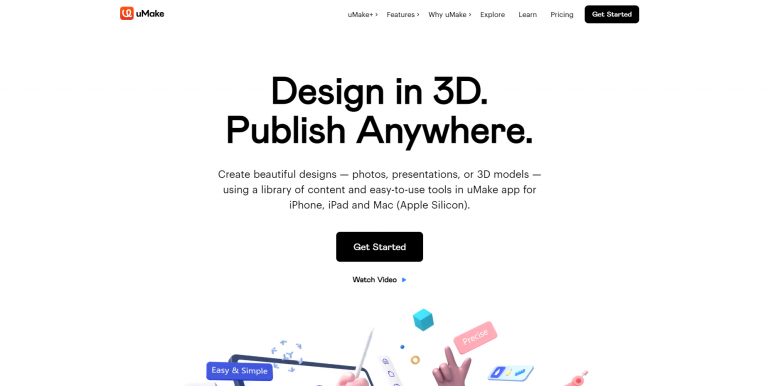The image captures a screenshot of a web page with a focus on promoting the YouMake app. The background is predominantly white with black text. The header of the page prominently displays the YouMake logo in red, positioned at the upper left-hand corner, followed by the name "YouMake." 

Centered on the page is a prominent heading that reads: "Design in 3D, Publish Anywhere." Beneath this, a detailed description highlights the app’s capabilities: "Create beautiful designs, photos, presentations, or 3D models using a library of content and easy-to-use tools in YouMake app for iPhone, iPad, and Mac, Apple Silicon." 

A noticeable black tab labeled "Get Started" is presented below this text, providing an easy call-to-action for users. Additionally, there is an option to watch videos for further understanding of the app, located just below the main description.

At the top of the page, various pull-down menus are accessible with choices like YouMake Plus, Features, Why YouMake, Explore, Learn, Pricing, and Get Started, offering a seamless navigation experience.

Towards the bottom of the page, the design is complemented by illustrative images of hands, buttons, and cubes, creating a dynamic and engaging visual appeal to enhance the thematic focus on 3D design.